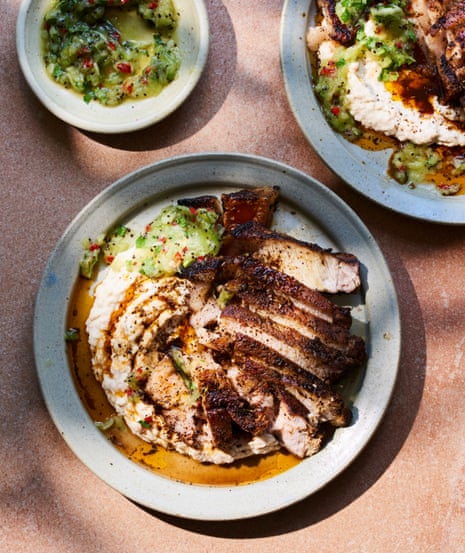The photograph features three light gray dishes set against a brick red background. The prominent dish, positioned slightly left and below the center, showcases beautifully sliced, browned meat that appears to be either chicken or pork, fanned out to reveal its white inner parts. Adjacently, on the left side of the plate, there's a generous serving of mashed potatoes with a drizzle of brown gravy. A small dollop of green sauce is placed at the top of the plate, adding a vibrant touch. Above and to the left, a small white bowl contains more of the green sauce. In the top right corner, partially visible, is another dish mirroring the main one with similar arrangements of browned meat and mashed potatoes, topped with green sauce. The top left of the image is slightly cut off, revealing a smaller plate with a green and red mixture that could be another variety of sauce or a soupy item.